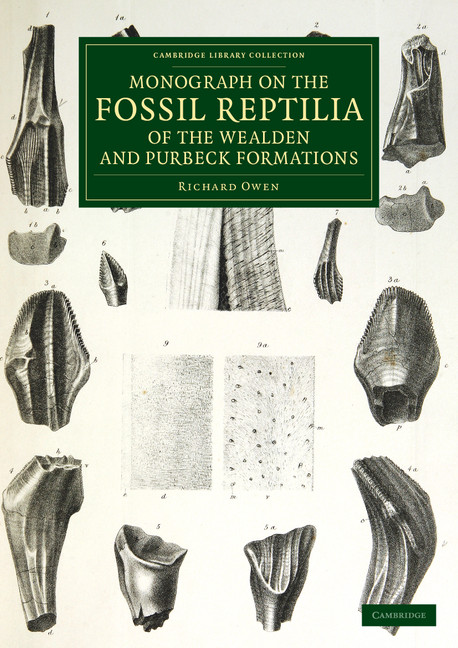The image appears to be a detailed illustration from an old book, likely from the Cambridge Library Collection, titled "Monograph of the Fossil Reptilia of the Wealdon and Purbeck Formations" by Richard Owen. The centerpiece of the image is a green rectangular banner at the top, featuring yellow text that reads "Cambridge Library Collection" and "Monograph of the Fossil Reptilia of the Wealdon and Purbeck Formations," followed by a thin horizontal line and the name "Richard Owen." Surrounding this banner are various fossil illustrations, all in different shapes and sizes, and presented in a grayish sketch style on a cream or grayish-pink background. The fossils are carefully arranged and numbered, each with distinctive curves, grooves, and patterns. At the bottom right of the image, there's a small green rectangle with yellow text that says "Cambridge." The page appears to be a meticulously drawn plate from a scholarly book, showcasing between 10 to 20 fossils of diverse forms, likely from the formations mentioned in the title.